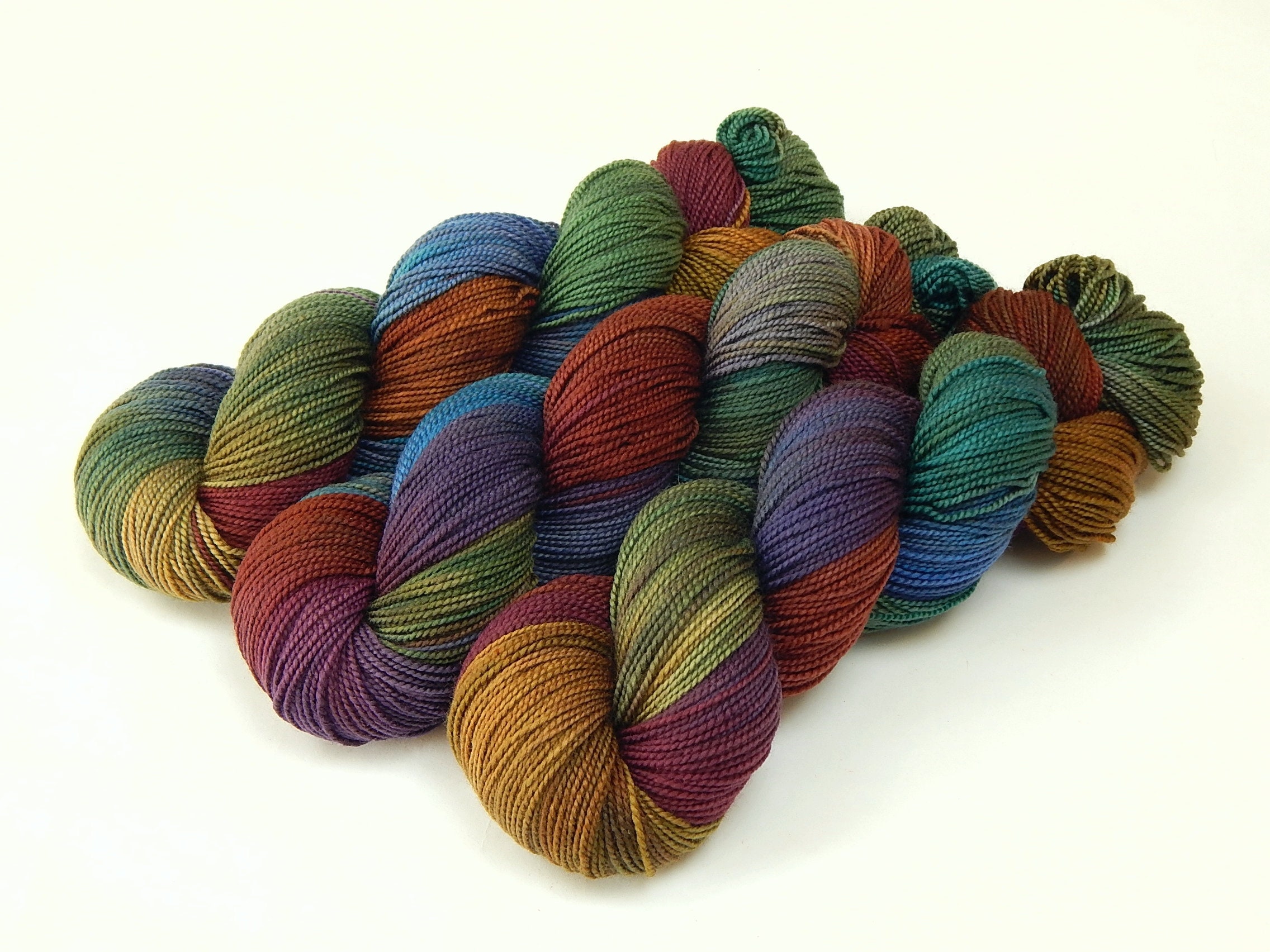The image depicts three intricately twisted bundles of fine, multicolored yarn, each resembling braided or knotted shapes akin to tiger tail doughnuts. Set against a plain, cream-colored background with a subtle shadow cast by the yarn, the bundles are uniform in size and wrapping style, showcasing a vast array of intertwined colors. The yarn features an earthy yet vibrant palette, including shades of yellow, green, maroon, purple, blue, teal, gold, burnt orange, and reddish hues. The colors smoothly blend into one another, with instances of yellow merging with green and purple interspersed with pink. The overall appearance of the yarn suggests a soft, thin texture, suitable for finely detailed knitting projects.